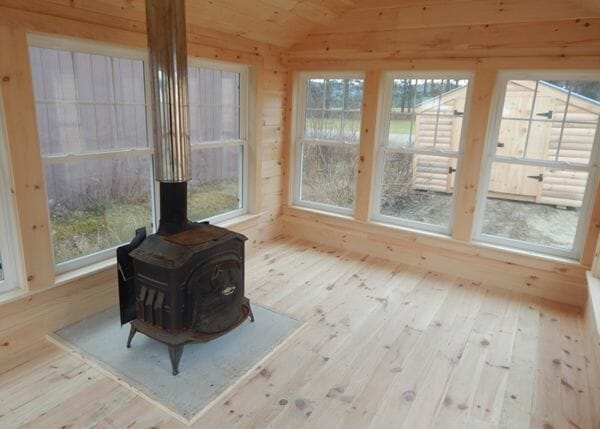The photograph captures the interior of a nearly empty room in a house, characterized by its completely exposed, nude wood surfaces, including the walls, ceiling, and floor. The room appears to be in a newly renovated state, with the wood possibly freshly sanded. Central to the image is an old-style, black wood-burning stove situated on the left side of the room. This stove stands on four legs, is made from cast iron or steel, and connects to the ceiling via a shiny, silver pipe. Surrounding the space are five large, bare windows without curtains, which allow a view of a sparse yard, a road, and a small wooden shed or log cabin in the distance. The room feels expansive, with the only furnishing being the stove resting on a square mat, underscoring the raw and rustic appeal of the setting.